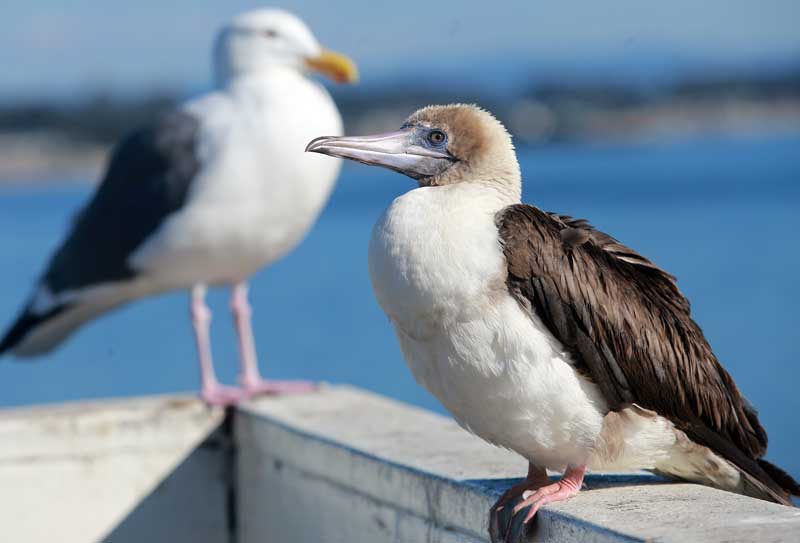This color photograph captures a detailed scene of two seabirds perched on a worn, gray stone ledge. The ledge has visible streaks and age marks, adding texture to the setting. In the foreground, there is a seabird with a grayish-brown, fuzzy head, adorned with both brown and white feathers. Its long, gray pointy beak and light-colored iris encircle its brown eyes with a hint of blue. Its underside is completely white, contrasting with its black wings, and it has notably short legs with long claws. This bird faces left, and its focus draws attention to its intricate details.

In the background, slightly blurred, stands a seagull. It has a white face, belly, and black wings with an orange beak. It is perched on the upper left corner of the ledge, facing right, displaying its long, skinny legs. The backdrop of the photograph shows a body of blue water with a distant shore lined with trees and a beach under a blue sky, creating a serene coastal ambiance.